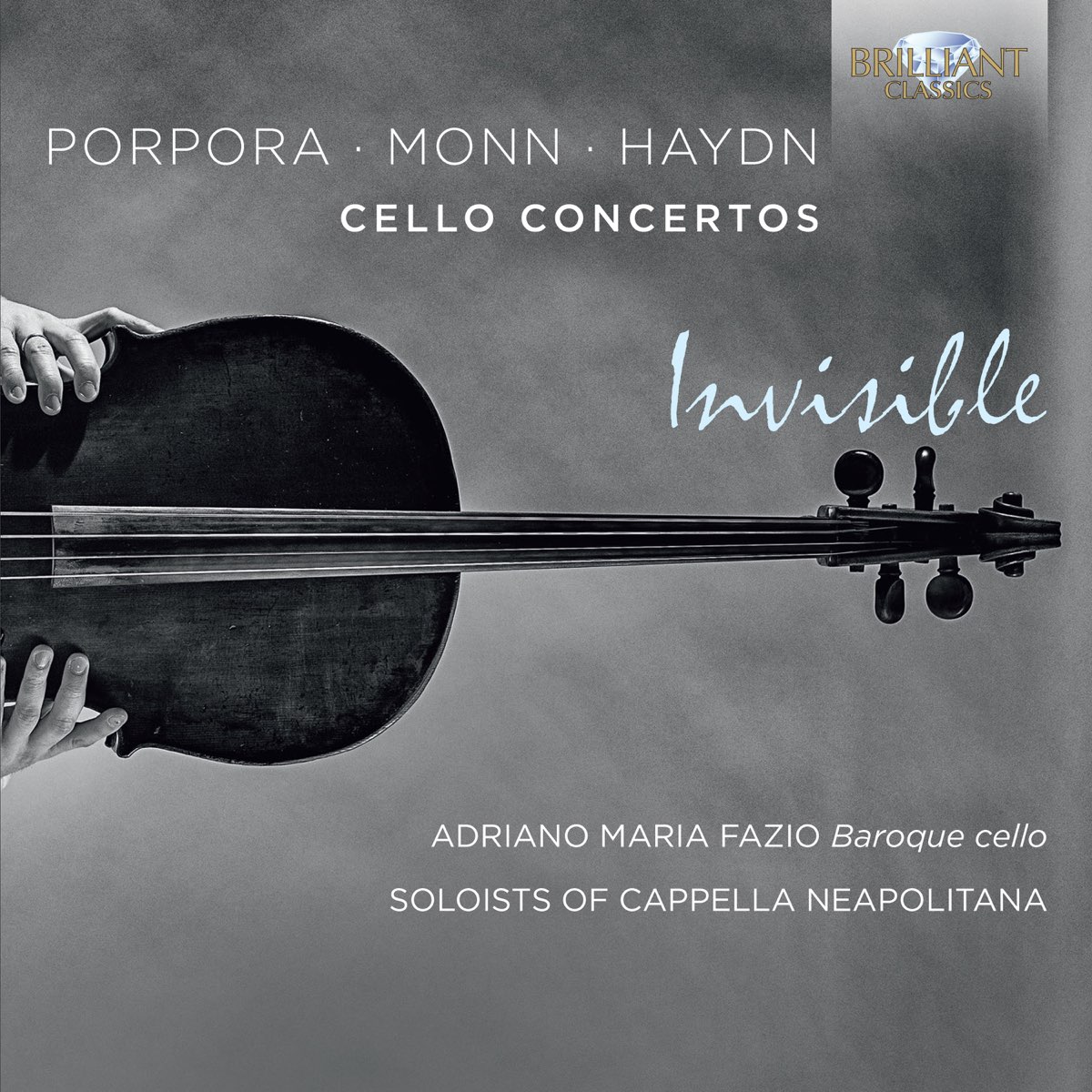This black-and-white photograph, likely an advertisement or promotional image for Brilliant Classics, showcases a detailed and finely captured representation of a violin or cello in a square format. The image is dominated by a horizontally positioned string instrument, with its body on the left and neck extending to the right. The instrument is being firmly held by two hands, one at the neck and the other at the body, emphasizing its classical charm and craftsmanship. The photograph utilizes a gradient gray background, adding depth and contrast to the scene. The text on the image is primarily in white and is arranged in a sophisticated layout. At the top, "Porpora • Mon • Hayden" is boldly displayed, followed by "Cello Concertos” in smaller but equally bold text. The artist's name, "Adriano Maria Fazio, Baroque Cello," is inscribed near the bottom right, along with "Soloists of Capella Neapolitana." A distinctive feature is the light blue italicized word "Invisible,” overlaying the right side of the instrument. Additionally, a gray rectangle in the top right corner with a shiny diamond illustration and gold text reads “Brilliant Classics,” lending an elegant touch to the promotional design.